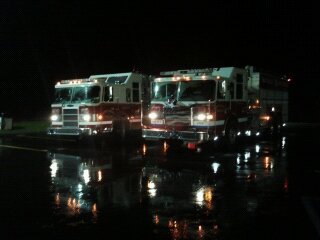This is a square, color photograph taken at night, showcasing two fire trucks positioned near a body of water. The nighttime setting casts a black backdrop, making the brightly lit fire trucks the focal point. Both fire trucks, primarily red with white upper sections, have their headlights and other lights turned on, illuminating the scene and creating vivid reflections on the wet ground or water surface in front of them. The fire trucks, although similar in appearance, show slight differences in their front grills, with one having a wider grill compared to the other. The image, likely taken with a high-quality camera, emphasizes the symmetrical reflection of the lights on the slick surface, adding a striking visual element. Despite the overall darkness, the lights from the fire trucks ensure they stand out sharply against the black sky, suggesting a professionally taken photograph potentially for a fire company's promotional use.